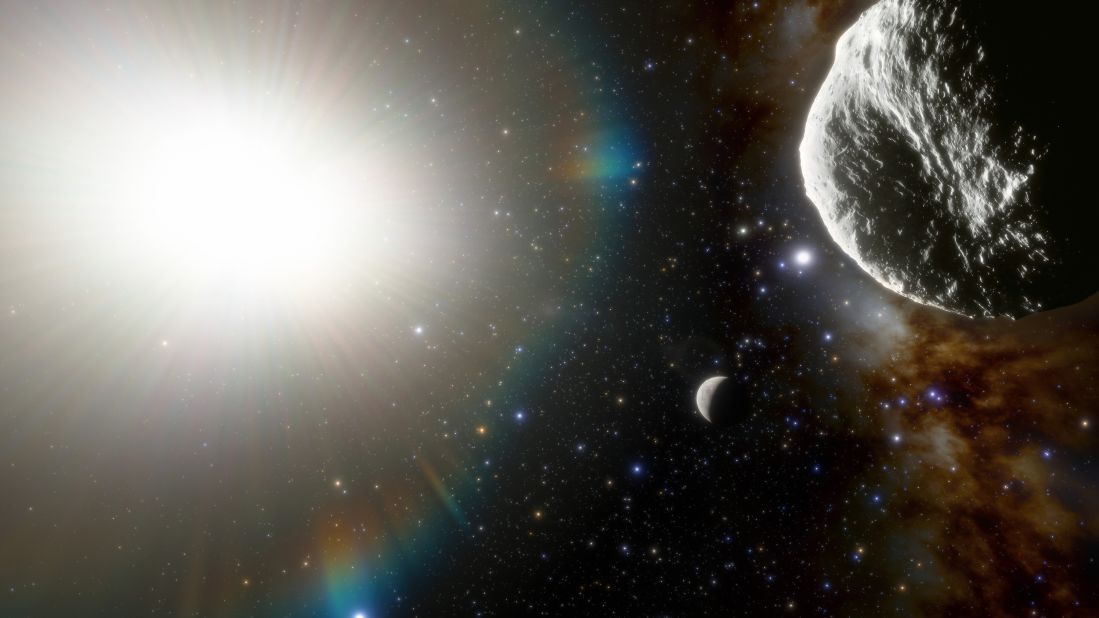In the vast expanse of the universe, a myriad of celestial bodies present a mesmerizing scene. Against the pitch-black backdrop studded with distant stars and planets, the partially shadowed moon reveals its enigmatic contours. Dominating the left side of the image, a radiant orb blazes intensely, filling half the frame with its brilliant light. To the right, an irregularly-shaped planet with a rugged, rocky surface stands out, part of it shrouded in darkness. Below this planet, wisps of cloudy, white fog drift, adding a layer of mystique to the cosmic tableau.